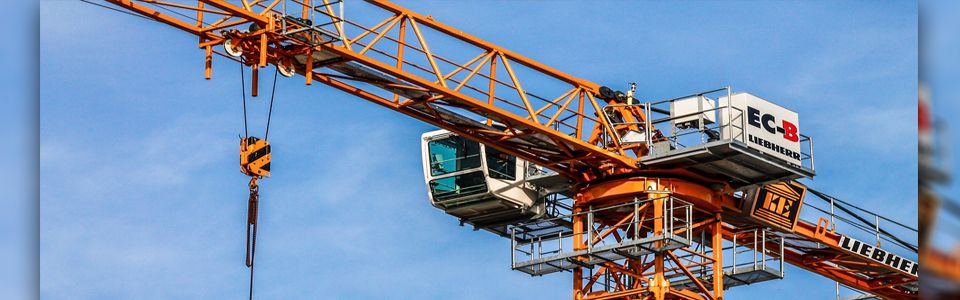This outdoor photograph captures a large horizontal construction crane in active use against a clear, bright blue sky accented with soft white clouds. Dominating the skyline, the crane extends diagonally with robust, thick yellow bars spanning across the image. There is a prominent white section on the crane, which bears the labels "EC-B" and "LIEBHERR" in black lettering, indicating the manufacturer's identification. Additionally, a small white compartment with glass windows, presumably for operating the crane, is visible on the crane’s side. A pulley system with cords hanging down can be spotted on the left side of the crane. This piece of heavy construction equipment is engaged in moving materials, possibly concrete or bricks, to aid in building a structure at the construction site. The overall scene is set under a clear, sunny, and bright sky, emphasizing the crane’s towering presence and active role in the ongoing construction work.